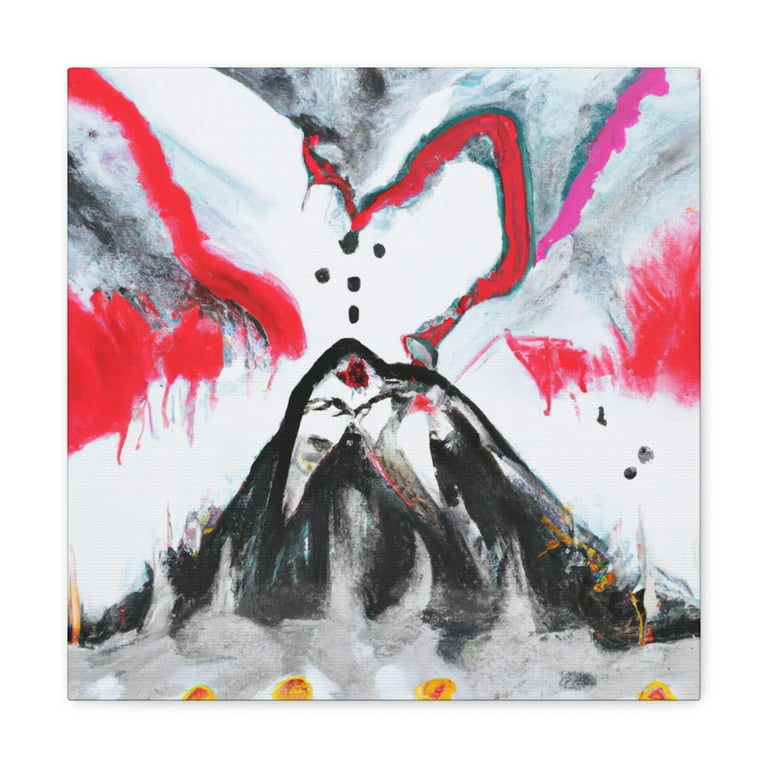This is an abstract painting featuring a vibrant and dynamic interplay of colors and forms. Dominated by hues of yellow, gray, black, red, pink, and white, the composition evokes a mountainous landscape with a prominent red streak extending upwards, suggesting volcanic activity. The sky echoes this tumultuous energy with streaks of red, blue, greenish-blue, black, and gray. Central to the piece are two abstract figures with black hair, their heads touching, symbolizing an intimate connection amidst chaos. Their faces hint at human features, yet remain non-realistic. Scattered around these figures are red marks, black dots, and diffused pink and orangish areas. Along the bottom, four yellow circles with orange centers add a rhythmic element. The overall texture of the painting is characterized by harsh brushstrokes, zigzag motions, and almost smoke-like, diffused paint, creating a sense of movement and depth. In the center, an 'X' shape stands out, almost like a void amidst the bustling array of forms and colors.